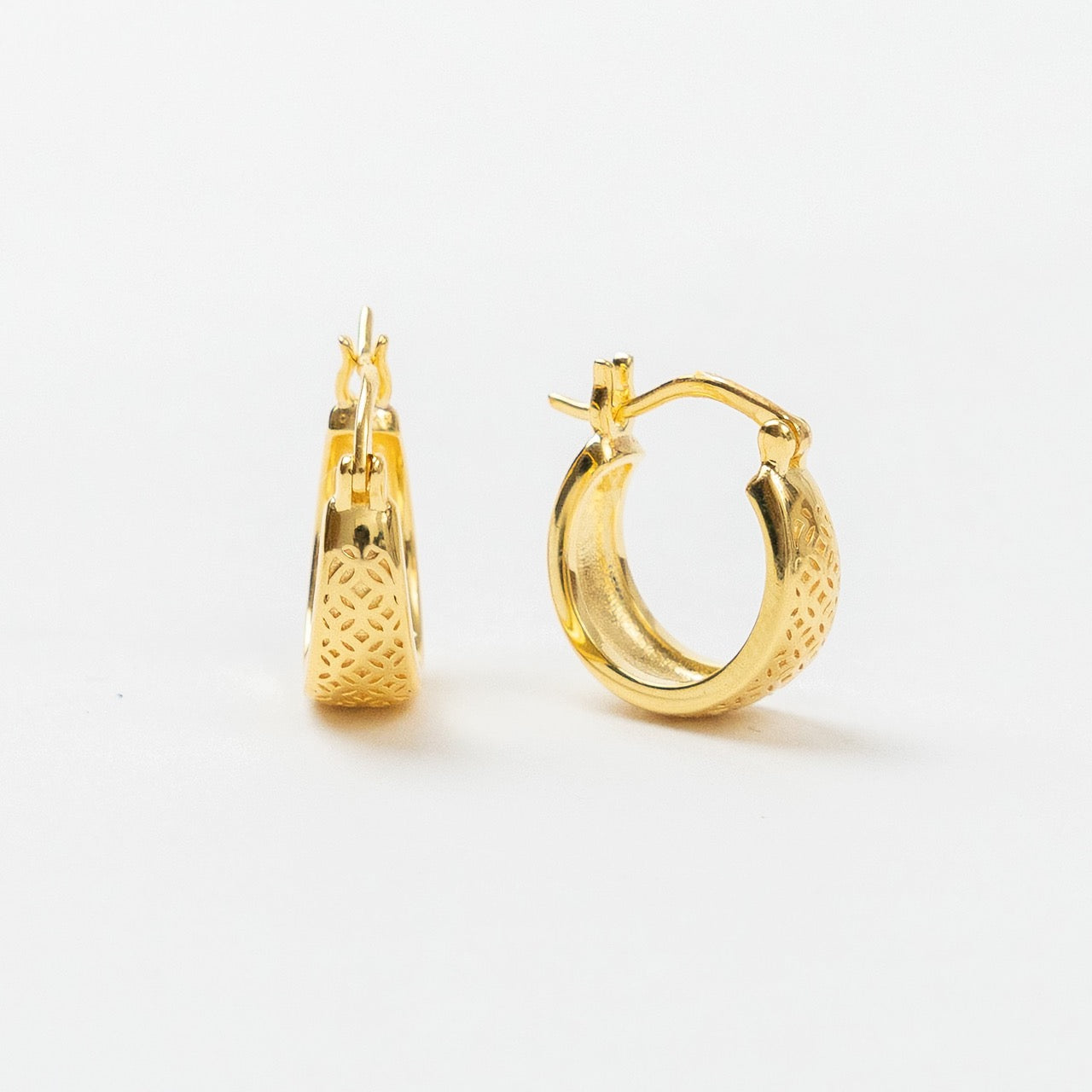The image is a color photograph showcasing a pair of elegant gold hoop earrings set against a white background. Both earrings feature a circular design with intricate interwoven Celtic or lattice-style engravings that adorn their outer circumference. The earring on the left is displayed head-on, highlighting its circular form and simple clasp mechanism at the top. Meanwhile, the earring on the right is angled at about 45 degrees, providing a clear view of its side profile. The clasps are U-shaped, designed to fasten securely. The earrings widen slightly towards the bottom, adding to the intricate detailing. The photograph captures the earrings with a mix of shiny and matte finishes, emphasizing the texture differences between the engraved exterior and plain interior. The light source, coming from the upper left, casts soft shadows and reflections, adding depth and highlighting the earrings' gold sheen. This close-up image provides a detailed view perfect for appreciating the craftsmanship of the jewelry.